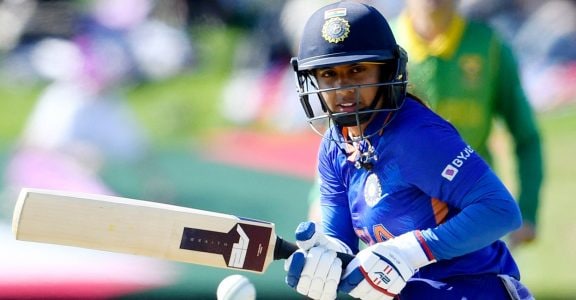The image captures an intense cricket match featuring a woman ready to bat. She is dressed in her team's bright blue uniform, adorned with orange numbers, although the exact number is unclear. She sports a black helmet with a protective face cage and a circular sports emblem on top. Her focused gaze is fixed on the incoming white cricket ball as she grips a light sandy wooden bat with a brown bottom and handle. Her hands are covered with white gloves embellished with blue and red details. In the blurred backdrop, there's a person in a green long-sleeve shirt with a yellow collar, possibly an umpire or an opponent. The field stretches out behind her with a mix of white, blue, green, and hints of pink and red.